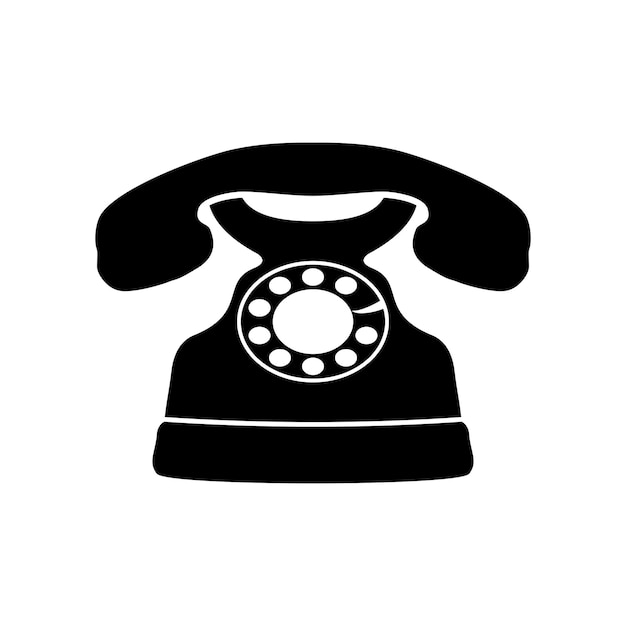This image depicts a basic computer-generated illustration of a classic, old-fashioned black rotary telephone, set against a completely white background. The telephone, almost a silhouette due to its solid black color, features a receiver resting on top of the handset, which is slightly curved upwards where the phone would hang up. The rotary dial, positioned centrally, is outlined in white and includes ten white finger holes used for dialing. There's a notable small white stopper at around the two o'clock position on the dial that prevents over-rotation. The base of the telephone is wider than the top, with a distinct horizontal white line near the bottom, separating the rotary dial from the telephone's base. This stark, unshaded image emphasizes the vintage design of the telephone, presenting a clear contrast between the black phone and its white background.